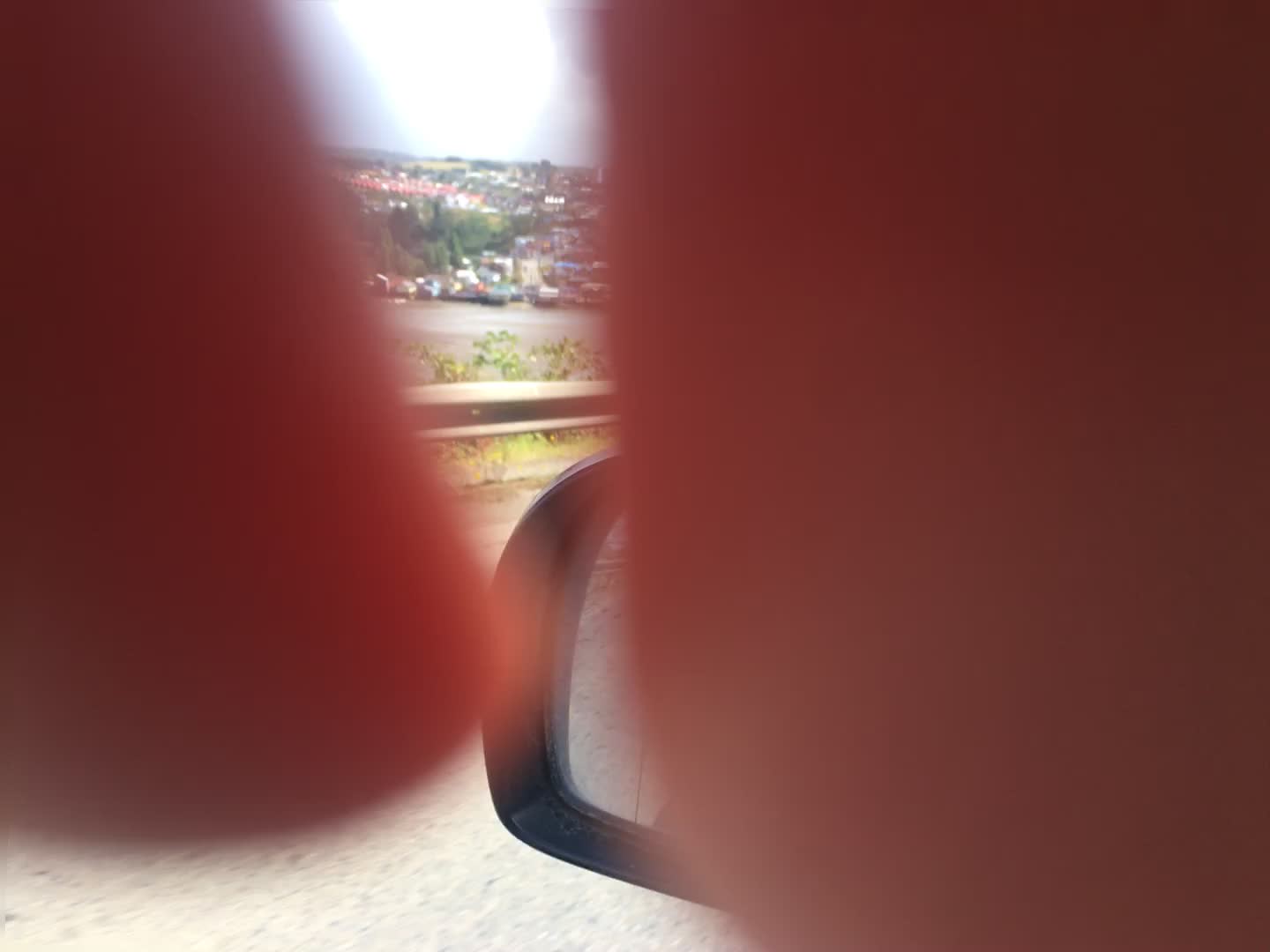This outdoor photograph, taken from inside a vehicle, is largely obscured by two pinkish fingers covering a significant portion of the camera lens, particularly the left and right sides. Through the gap between the fingers, one can discern a black driver's side rearview mirror and a partial view of the highway below. Beyond the road lies a grassy area with a metal guardrail. In the distance, there's a gently sloping hill adorned with trees and houses, some of which are part of a residential street that is faintly visible. Further away, there is a cityscape featuring buildings and vehicles, with some green shrubbery interspersed. A stretch of sky frames the distant horizon, completing this obstructed yet detailed scene.